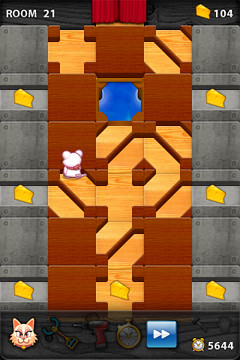The image depicts a pixelated platform game designed for a Java-based cell phone. At the top, "Room 21" is displayed in white text on the left, with "104" and a yellow cheese icon on the right. The game screen features a vertically-oriented maze with seven cheese cubes scattered throughout. The maze is dark brown with gold accents and bordered by gray platforms. The objective appears to involve navigating a small mouse character to collect cheese while avoiding obstacles. In the lower left corner, there is an array of icons, including a dramatic-eyelashed face resembling a cat or bunny, a claw tool, an electric screwdriver, a stopwatch, a fast-forward button, a small hammer, and an old-fashioned alarm clock with the white text "5644" next to it. The bottom right corner of the screen shows a blue square with two arrows pointing to the right. Above these icons, a blue circle possibly representing a body of water is visible. The top of the screen also features red curtains, adding a theatrical touch to the game's design.